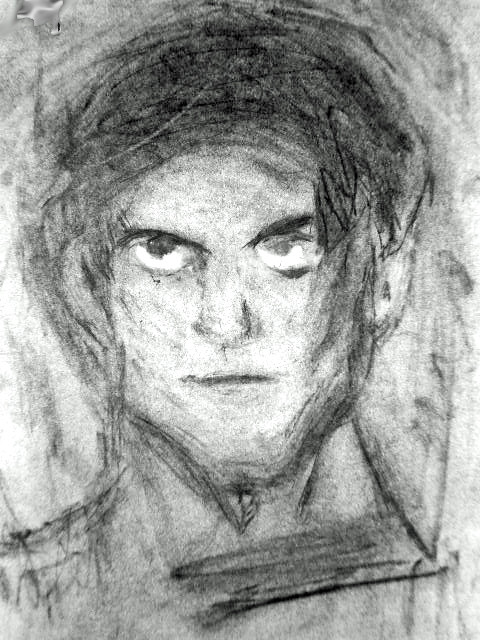This image is a vertically oriented photograph or scan of what appears to be a hand-drawn sketch on white paper. The artwork features a detailed, highly textured black-and-white sketch of a man, most likely executed with a black pencil or charcoal, giving it a somewhat scratchy appearance with various shades of gray for shading. The man in the sketch has straight, black hair that droops just above his ears, light colored skin, and distinct black eyebrows. His eyes, white with black pupils, are glancing upward, adding an expressive element to his face. His mouth is drawn in a neutral, horizontal line, contributing to his overall determined and confident demeanor, though he also appears slightly upset. The character has a chiseled jaw and the upper portion of his neck is visible, with subtle sketch lines and shading surrounding his form, adding depth and texture to the monochrome piece.